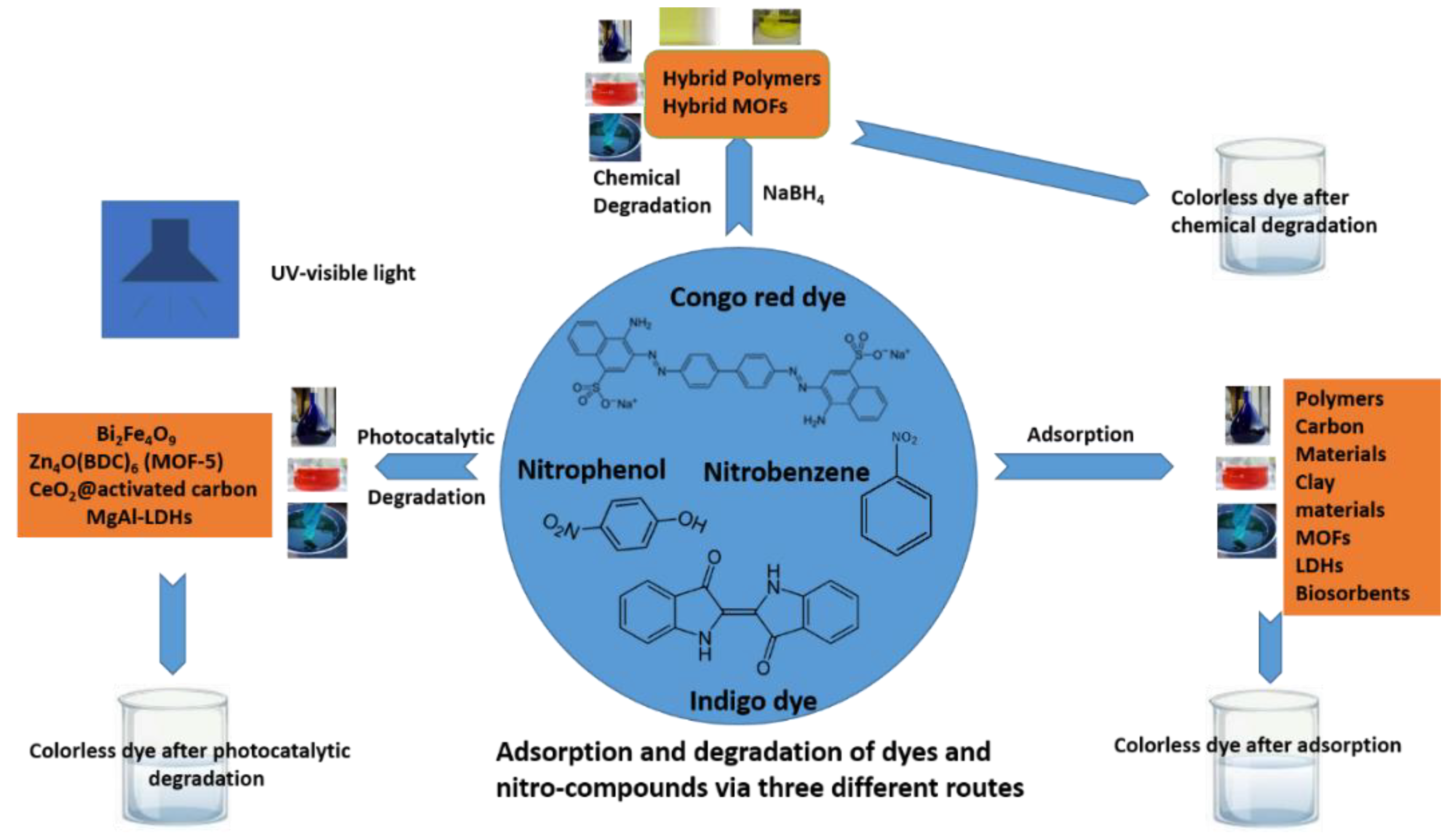This detailed infographic, set against a white background, visually represents complex chemical and biological processes in a flowchart format. At the top, various chemicals are depicted, including hybrid polymers and Metal-Organic Frameworks (MOFs), with a focus on chemical degradation. 

Central to the image is a large blue circle featuring molecular structures and labels for various compounds, such as Congo Red Dye, Nitrophenol, Nitrobenzene, and Indigo Dye. Molecular diagrams accompany these labels, displaying specific bonds like O2N and OH. Beneath this blue circle, there is text stating "Adsorption and degradation of dyes and nitro compounds via three different routes," from which emanate three distinct blue arrows.

The first arrow leads to a section labeled "Photocatalytic Degradation," marked by an arrow to the left of the central blue circle. A notable detail here includes an orange box displaying chemical formulas and a blue box at the top with "UV visible light." The process concludes with "Colorless dye after photocatalytic degradation" at the bottom of the orange box.

On the right side of the flowchart, another orange box, marked with additional chemical formulas, depicts two beaker images. The top beaker is associated with photocatalytic degradation, while the bottom one represents "Colorless dye after adsorption."

Overall, the infographic meticulously illustrates the pathways and chemical processes involved in the degradation and adsorption of various dyes and nitro compounds through photocatalysis, chemical degradation, and adsorption.